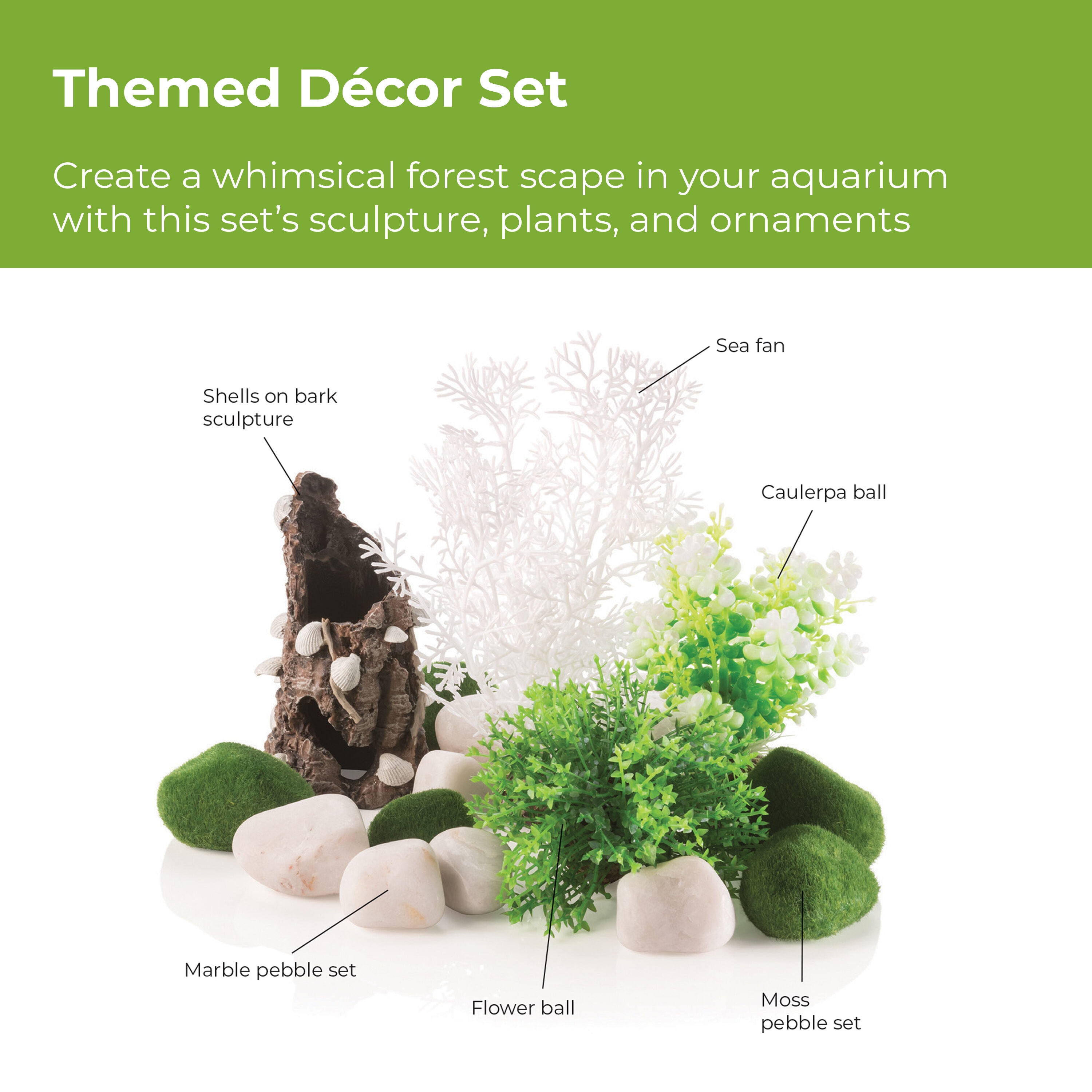The advertisement for aquarium supplies features a green rectangular text box at the top, with white font reading "Themed Decor Set." It invites viewers to "Create a whimsical forest scape in your aquarium with this set's sculpture, plants, and ornaments." Below this text, a photograph showcases the various components of the set, each labeled with their names. The items include a "Shells on Bark Sculpture," resembling a hollow tree stump adorned with shells; a white "Sea Fan" coral; a green "Caulerpa Ball" plant; a "Flower Ball," another green plastic plant; and two types of pebbles: the "Moss Pebble Set" with green, moss-textured pebbles, and the "Marble Pebble Set" featuring polished white pebbles. These components are arranged clearly, demonstrating the whimsical and decorative possibilities for an aquarium setup.